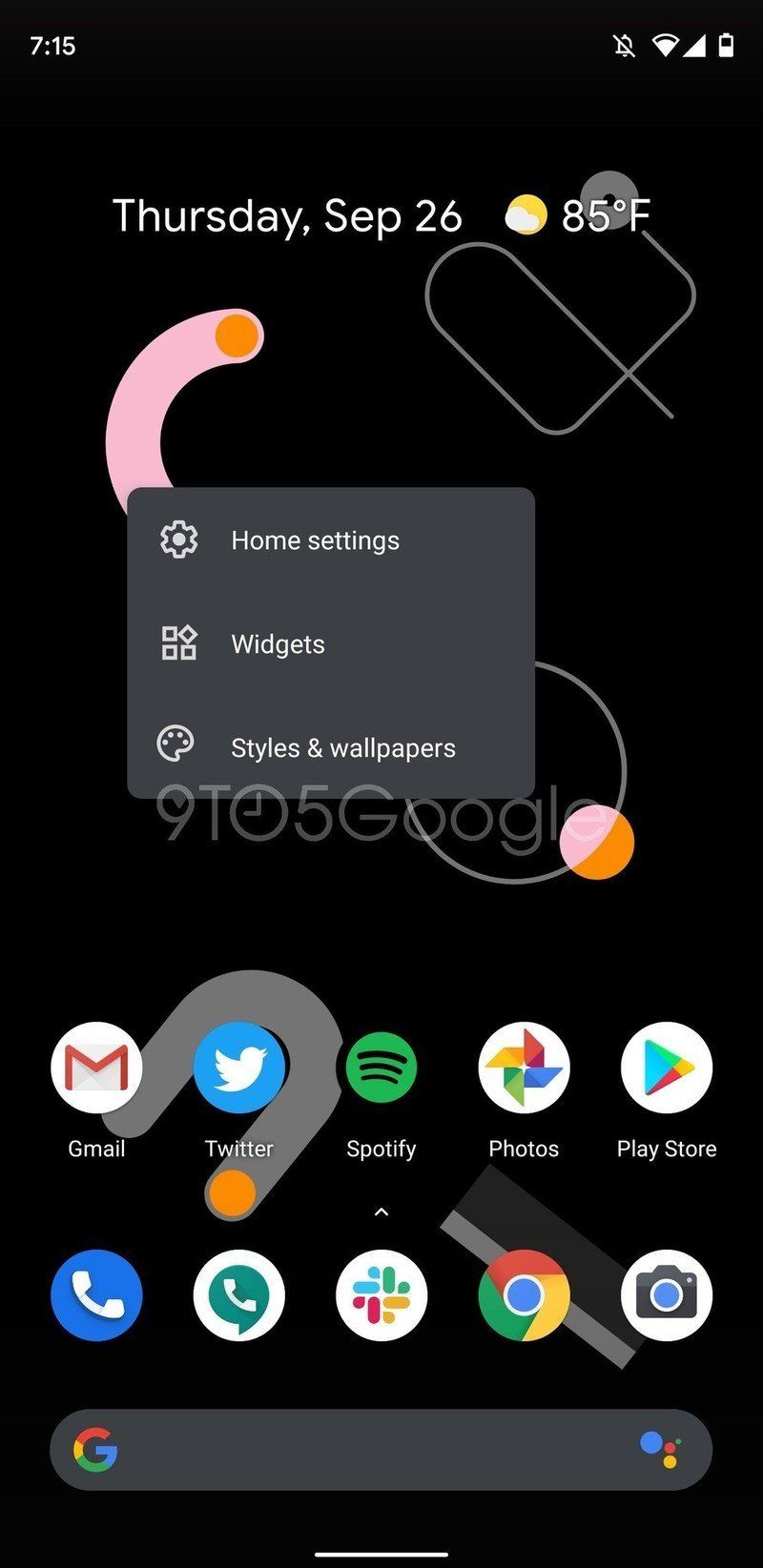A detailed screen capture of a cellphone display, captured at 7:15 AM with the battery indicator showing approximately 50% charge. The date is prominently displayed as Thursday, September 26th. The weather widget indicates a temperature of 85 degrees Fahrenheit with a partly cloudy icon. A pop-up menu is visible, offering options for home settings, widgets, styles, and wallpaper customization, likely triggered by a long press on the phone's background. In the lower portion of the screen, a watermark is visible, displaying the text "9TO5Google" with the "O" stylized as a clock showing 9 o'clock, suggesting that this image was published by a site or brand related to Google tutorials or technology guides.